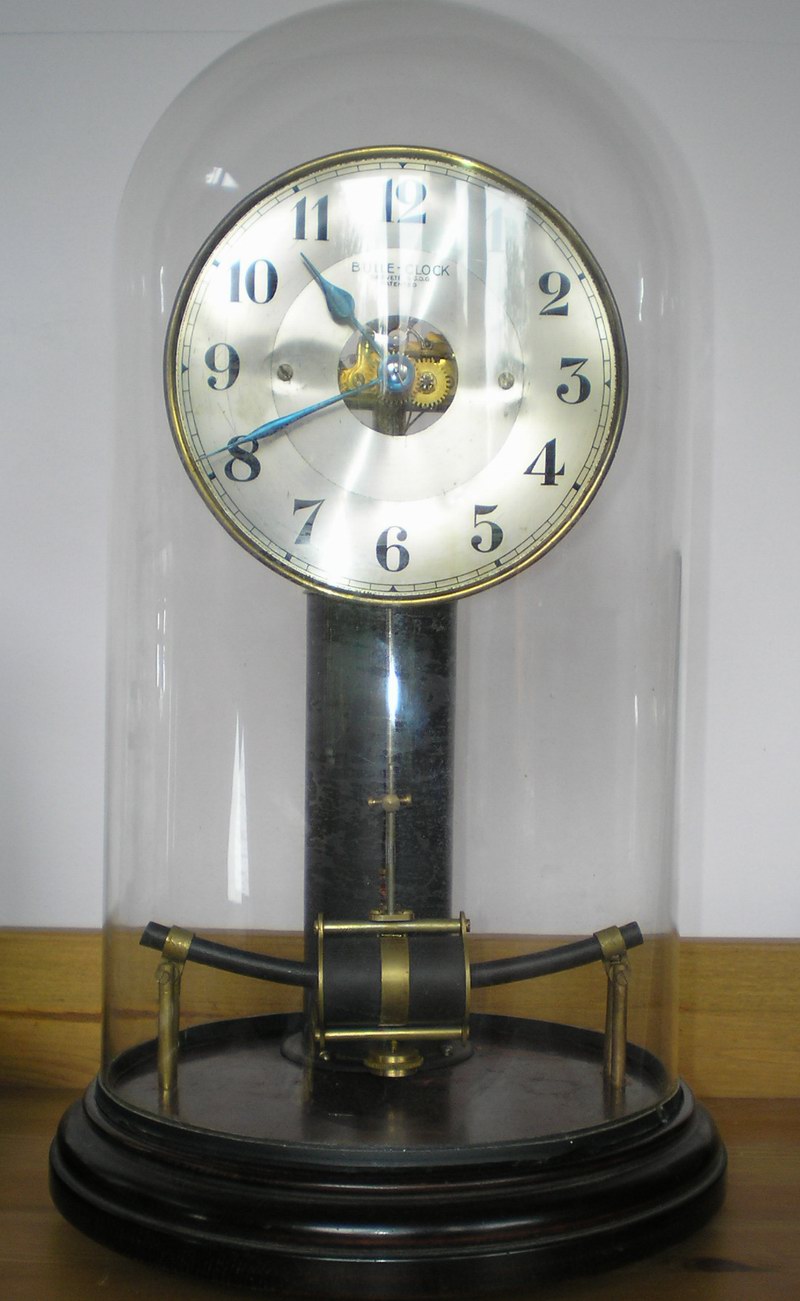The photograph showcases an up-close view of a vintage-style, antique desk clock encased in a clear glass dome shaped like a cylinder with an oval top. The clock, which exudes an old-style charm, is mounted on a black circular base and features a striking black tower that supports the clock head. The circular clock face is enclosed by a gold rim, and the large black numbers are easy to read. Intriguingly, a small transparent circle at the center of the clock reveals its intricate gold gears. The scene is set on a wooden table with a white wall in the background, highlighting the elegant simplicity of the clock’s design.